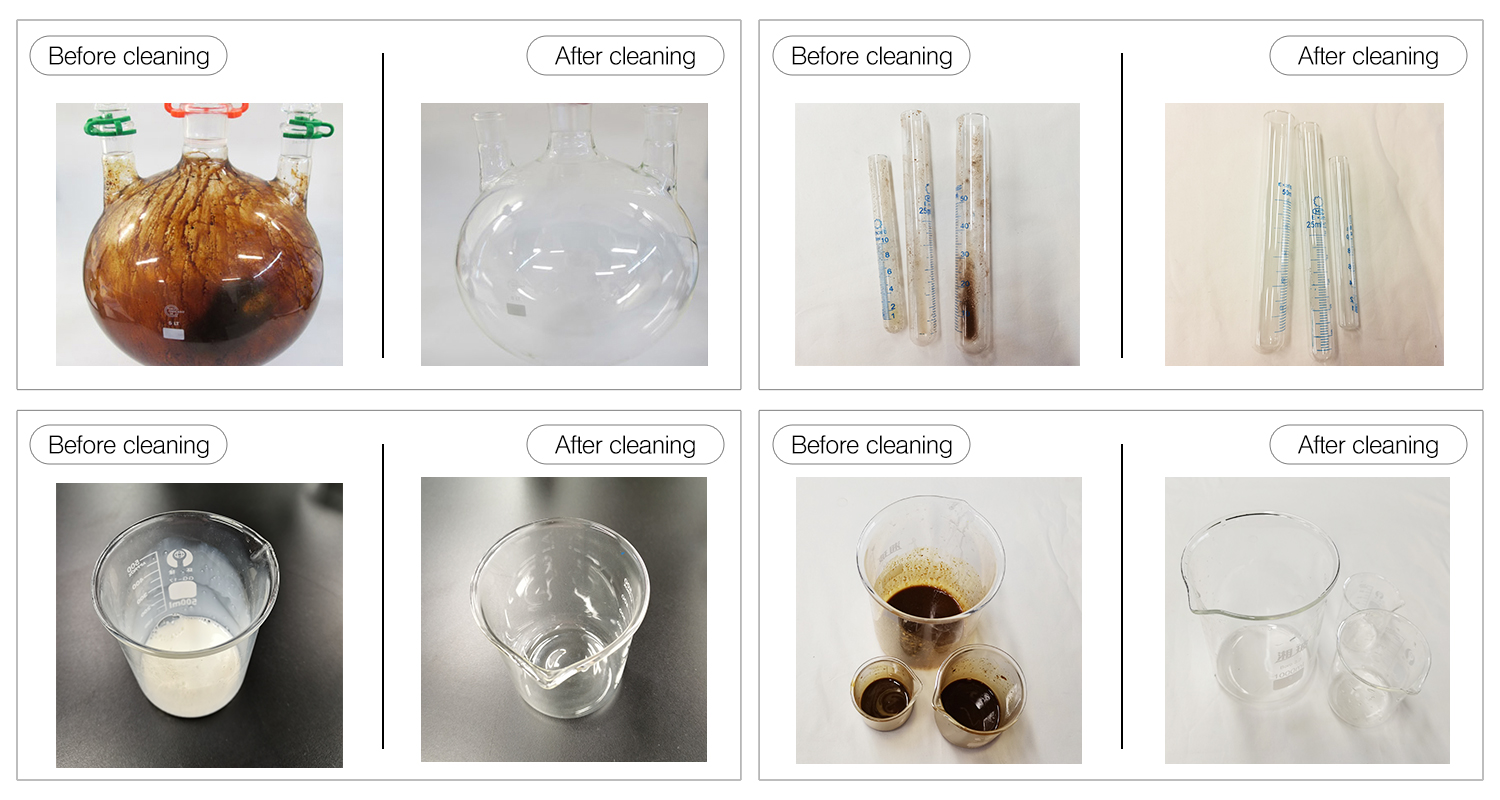The image is a horizontally aligned rectangular collage consisting of eight small pictures, separated by thin black borders. Each set of paired images depicts a Before Cleaning and an After Cleaning state of various laboratory glassware. 

In the upper left corner, the first pair showcases a dirty, brown flask labeled "Before Cleaning" and its sparkling, pristine counterpart labeled "After Cleaning." To the right, another pair follows the same theme with test tubes: the left image shows three murky test tubes, while the right presents them clean and clear.

The lower half mirrors this arrangement with two additional sets of Before and After Cleaning pictures. In the lower left corner, a beaker containing a milky white substance is shown "Before Cleaning," and next to it, a shining, empty beaker is labeled "After Cleaning." Finally, in the lower right corner, three beakers filled with dark brown liquid are depicted "Before Cleaning," and their gleaming, spotless versions are displayed "After Cleaning."

The image focuses on illustrating the dramatic transformation of laboratory glassware from dirty and grimy to impeccably clean through a series of detailed before-and-after comparisons.